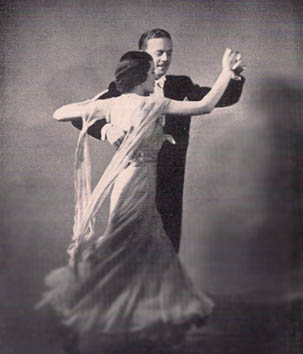In this vintage black-and-white photograph with a slight sepia tone, a young couple is captured mid-dance, reminiscent of the early 20th century, possibly the 1920s or 30s. The gentleman, facing the camera, sports a thin mustache and slicked-back dark hair. He is elegantly dressed in a tuxedo with a white shirt underneath, his left hand clasping the lady's right hand while his right arm wraps around her shoulder. The lady, viewed from behind, is adorned in a long, flowing white gown with an open back and delicate straps. Her flowing gown, accentuated by a long, swirling scarf, moves gracefully as she twirls, her left arm resting on the man's shoulder. The interplay of light and shadow in the dark, cloudy gray background enhances the poetic and romantic essence of their ballroom dance.